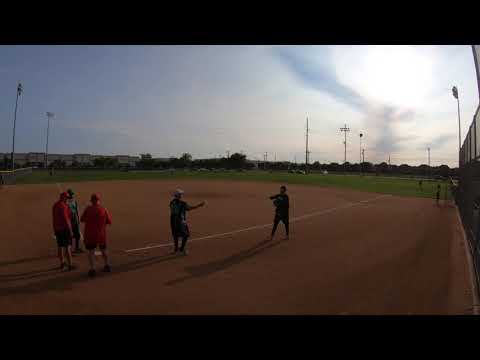A photograph captures a tranquil moment at dusk on a baseball field. The reddish-brown dirt of the baseball diamond contrasts with the green turf of the outfield. Clearly visible are the white chalk baselines, particularly one stretching towards the outfield. A group of five individuals congregates near this baseline, not actively playing but simply standing around. Among them, three wear red shirts and two are dressed in darker attire, possibly engaging with each other. The image, slightly blurry, shows the silhouettes of tall, unlit light posts and a chain link fence bordering the field on the right side. The sky above transitions from a dull blue to a cloudy white, hinting at the encroaching evening.